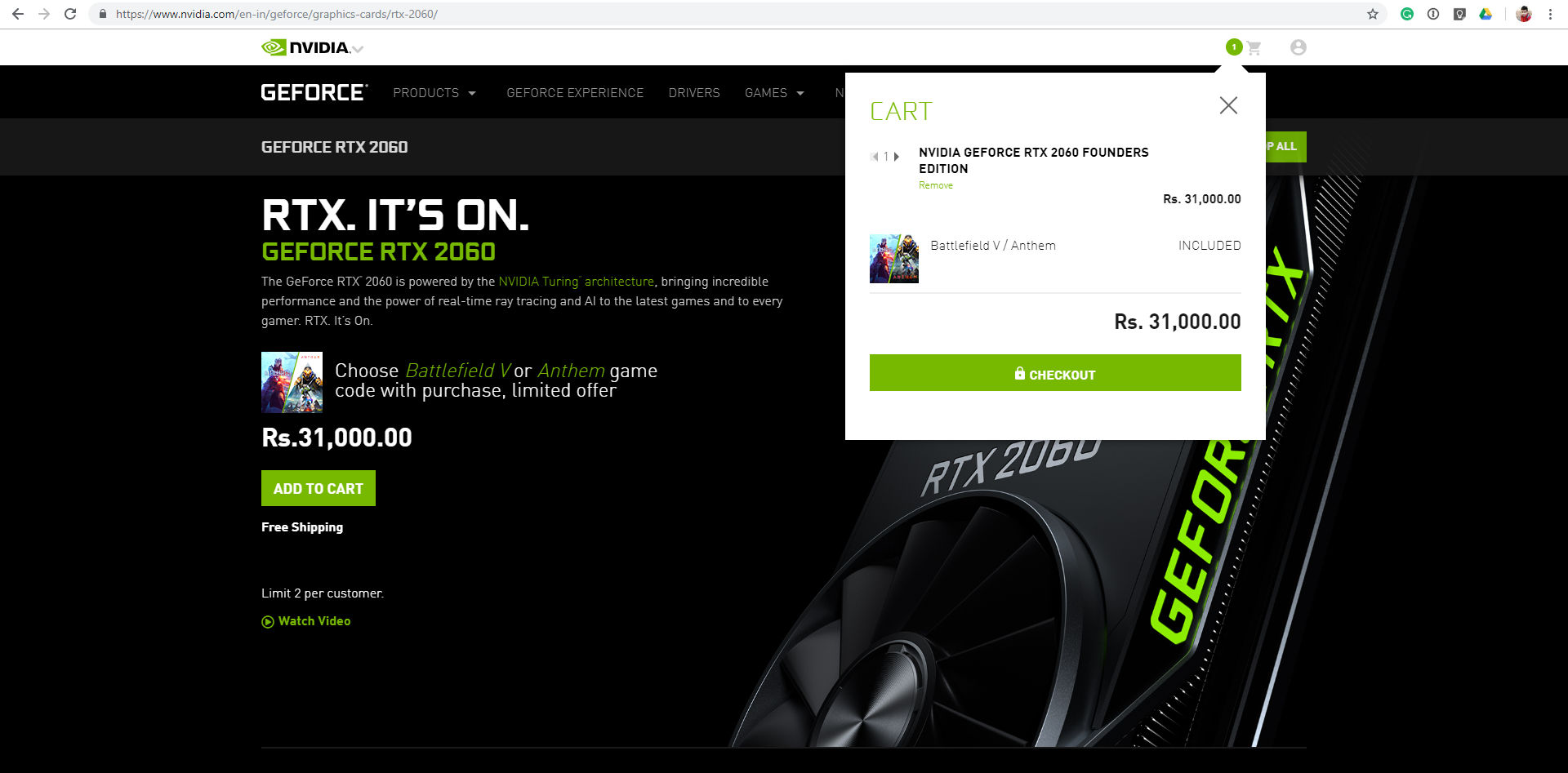**Screenshot Description: Detailed View of NVIDIA GeForce RTX 2060 Purchase Page**

This desktop screenshot captures a Chrome browser window open to the URL https://www.nvidia.com/en-in/geforce/graphics-cards/rtx-2060/. The page prominently features NVIDIA's branding, including the company logo and the word "NVIDIA" accompanied by a drop-down arrow. To the right, there is a shopping cart icon indicating one item inside.

**Shopping Cart Section:**
Below the main navigation bar, the shopping cart lists the item "NVIDIA GeForce RTX 2060 Founders Edition," which can be removed using the black 'X' icon. A small green hyperlink offers the option to remove the item. The price is listed as RS 31,000. Beneath the item description, it mentions that purchasing this product includes "Battlefield V / Anthem." The total price is again listed as RS 31,000, with a prominent green 'Checkout' button positioned below.

**Navigation and Product Information:**
On the left side of the predominantly black background, there is a navigation menu featuring tabs labeled "GeForce," "Products" (with a drop-down arrow), "GeForce Experience," "Drivers," and "Games" (with a drop-down arrow).

**Main Product Description:**
At the center of the page, the product featured is the "GeForce RTX 2060," further described with the tagline "RTX, it's on." The description elaborates that the GeForce RTX 2060 is powered by NVIDIA's cutting-edge Turing architecture, which offers remarkable performance and the power of real-time ray tracing and AI capabilities in modern games.

Crucial details, such as "NVIDIA Turing architecture," are highlighted in green, indicating clickable hyperlinks for additional information.